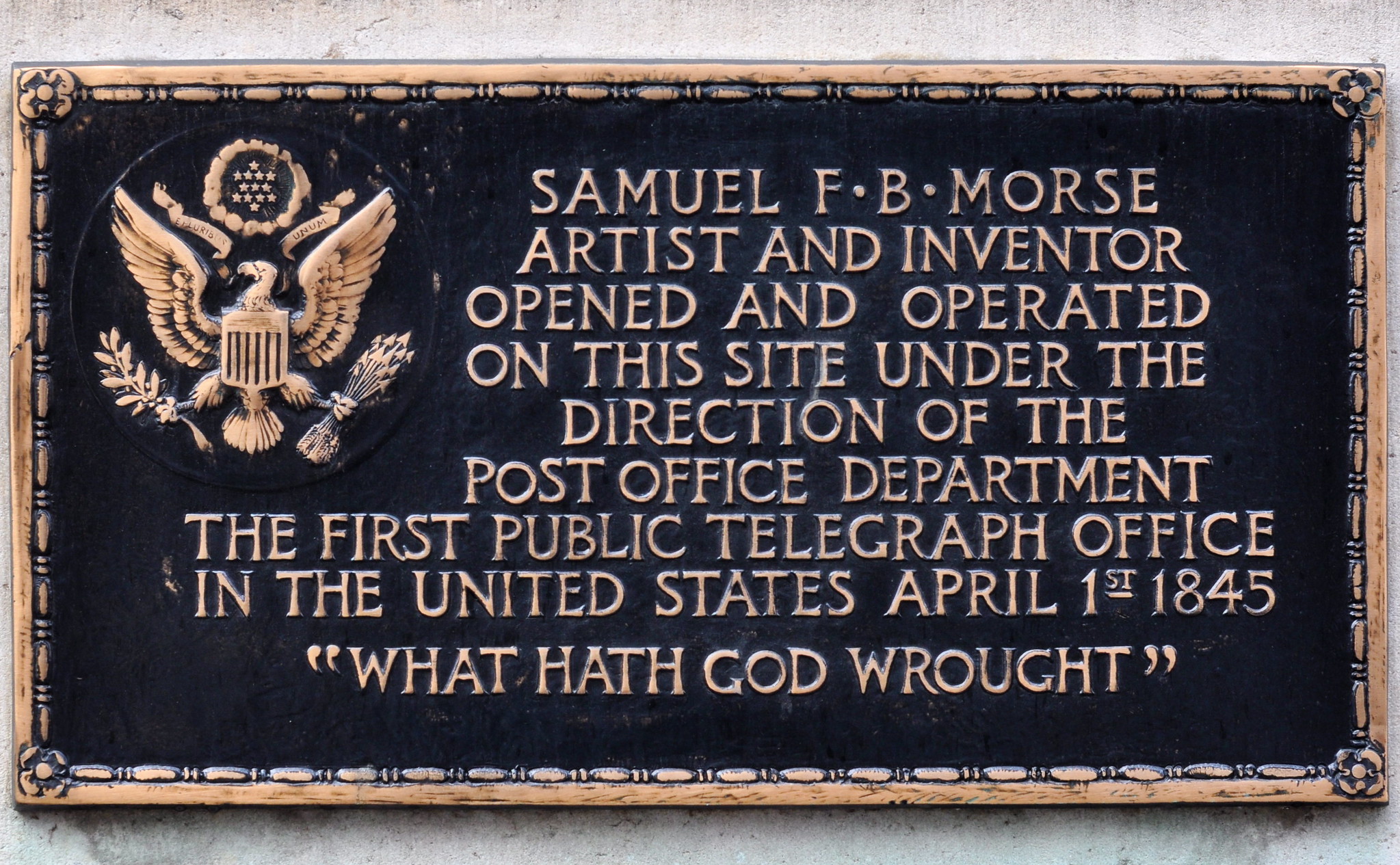The photograph, taken outdoors during the daytime, captures a six-inch-wide by four-inch-tall bronze plaque mounted on a stone wall. The plaque, a national United States historical marker, commemorates Samuel F. B. Morse, the illustrious artist and inventor. The rectangular plaque features a bronze or brass border with floral designs at each corner and a black background. In the upper left corner, there is a gold emblem of an eagle with a shield, holding laurel leaves in its right foot and a cluster of arrows in its left, with a circle of stars above. The plaque's inscription in raised gold print reads: "Samuel F. B. Morse, artist and inventor, opened and operated on this site under the direction of the Post Office Department, the first public telegraph office in the United States, April 1st, 1845." Below this is the first Morse Code message, "What hath God wrought." The monument marks Morse’s significant contribution to communication history, highlighting the first public use of the telegraph system.